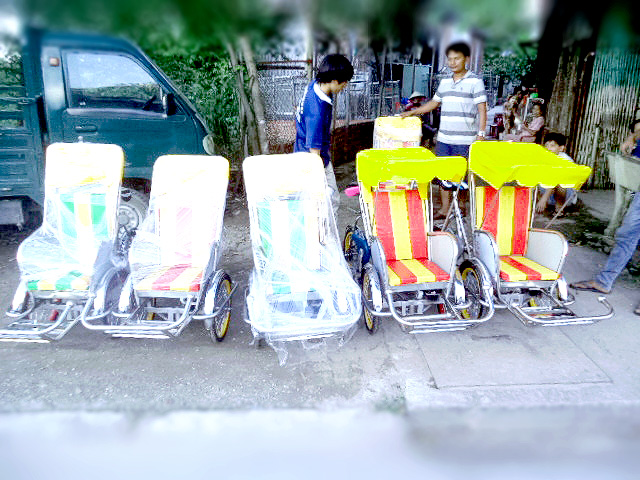A low-quality color photograph captured from inside a vehicle, probably a car or a bus, shows a bustling street scene that appears to be in Cambodia or Vietnam. The top and bottom edges of the photograph are blurred, likely due to a camera issue. Along the sidewalk, a series of rickshaw bikes are lined up. The three rickshaws on the left are heavily whited out with scarce detail, while two rickshaws on the right feature distinctive yellow and red stripes with yellow awnings. A bluish-gray pickup truck's front end intrudes from the left side of the image. Beside the truck, two men are standing; one wears a white-gray striped shirt, and the other a blue shirt with a white collar. Several other people are also present, albeit partially visible, some standing and some sitting. Behind the individuals, there are trees and gray metal fences, and in front of them are various chairs on wheels, possibly pedicabs, with striped patterns in red-yellow and green hoods. The background hints at an outdoor market area, with potential stalls or tables where items might be sold.